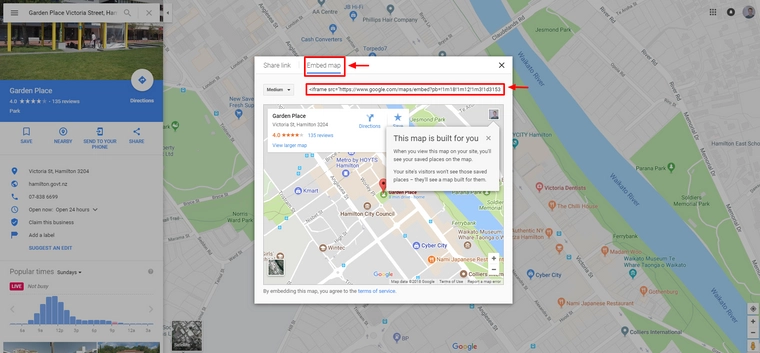In the image, there is an intricate overlay comprising various elements related to a map on a web browser. The central focus is a pop-up map, predominantly white, square-shaped, and located against a faint background map. On the right side of this pop-up is a distinct black "X," while the left side displays the text "shared link" in black, followed by "embed map." A red arrow and a red box highlight this segment, drawing attention to it.

A gray line horizontally traverses the image, separating sections. Below, another rectangular box encloses part of a web browser's address bar, although it appears blurred. Despite the blur, the text "https://www.google.com/maps" can be discerned, presumably starting with "https://" and featuring the letters "PS." This segment is also marked with a red rectangular box and a rightward-pointing red arrow.

Further below, the underlying map is visible once more, accompanied by another pop-up. This secondary pop-up, a gray rectangle with black text situated on the right side, reads: "This map is built for you. When you view this map on your site, you'll see your [...] places on the map." The word in the blank is unclear due to blurriness. Another notation, "Garden Place," is displayed on this pop-up, alongside an indication of "125 views." The detailed annotations and navigational guides emphasize specific functionalities and elements within an interactive map interface.